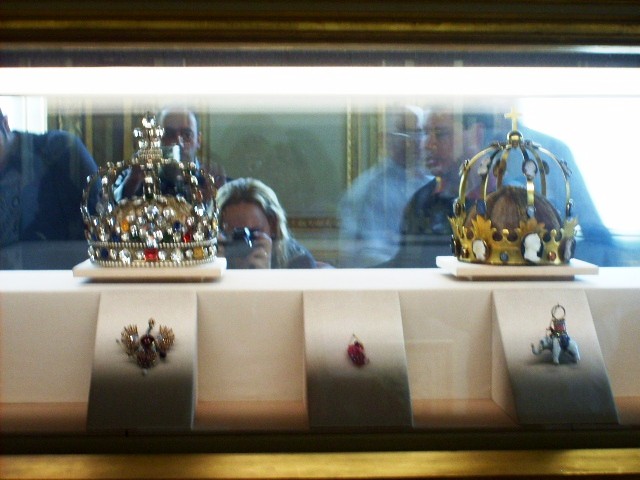In this rectangular photograph taken in a museum setting, we see a display case featuring two elaborate royal crowns, accompanied by three pieces of jewelry placed in front of them on individual stands. The crown on the left is heavily adorned with rubies, clear stones, and sapphires, and is topped with a gold cross. The crown on the right, simpler in design, showcases gold leaves and white cameos of busts around its base, with stones interspersed between the cameos. Among the jewelry, the piece on the far right is a white elephant adorned with additional shapes on its back, while the other two pieces are less discernible.

Visible through the glass behind the crowns are reflections of approximately five tourists, including a crouched individual. At the center, a woman with blonde hair is captured in the act of taking a photo, her camera held between her hands focused on the crown to the left. The background reveals blurred, ornate cream and gold walls adorned with frames. The display rests on a brown table or shelf, completing the setting.